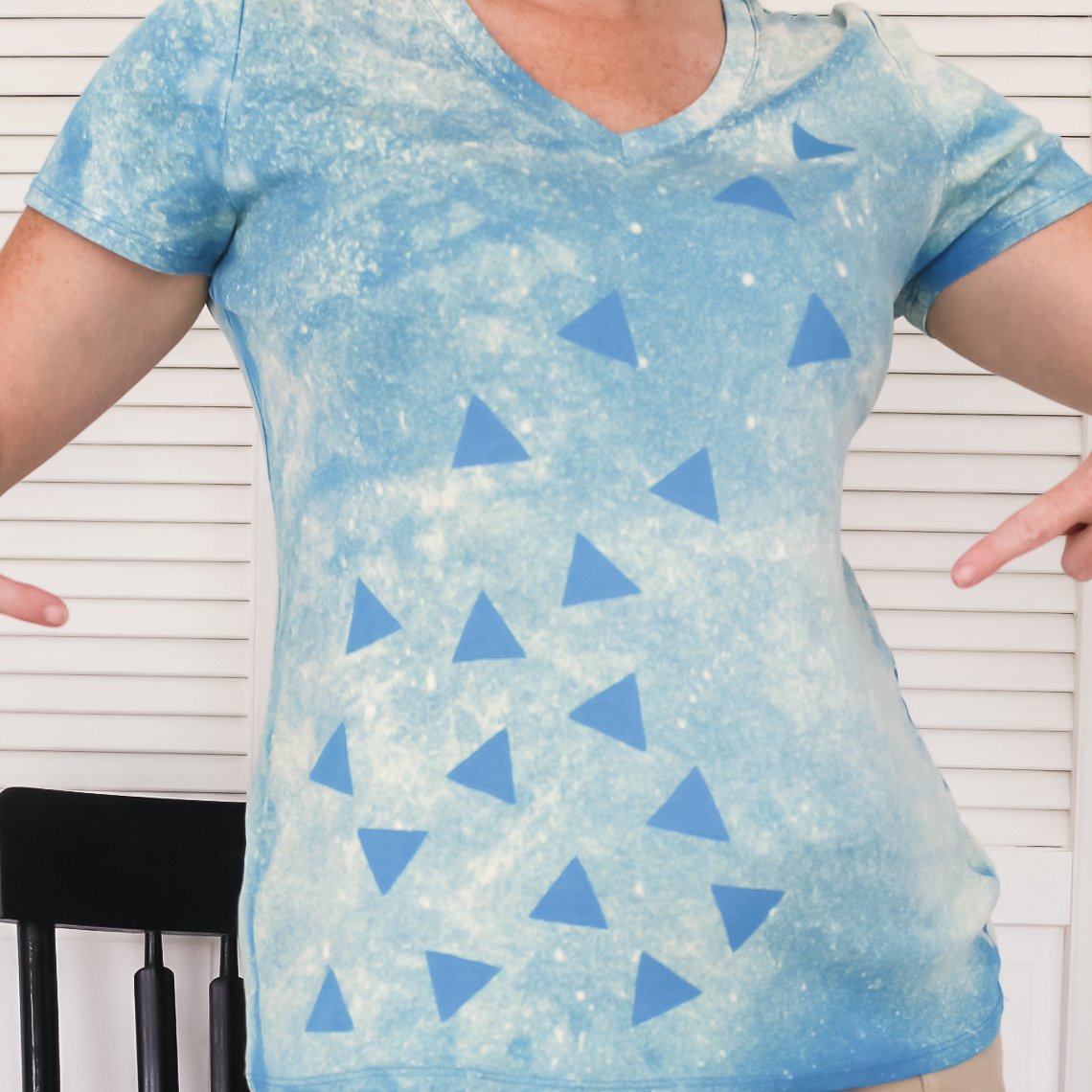The image features a cropped view of a Caucasian woman from the neck down to just above the hips, pointing at her shirt with both index fingers. The shirt is predominantly blue with white speckles, resembling a mixed paint effect. Overlaying this pattern are solid blue triangles that start from the lower left side of the shirt and ascend diagonally towards her upper right shoulder. The shirt is a fitted v-neck t-shirt with very short sleeves. The background consists of white house siding and a black wooden chair positioned to the bottom left. The woman appears to be of average build, possibly wearing khaki pants or shorts, although the view of her pants is limited.